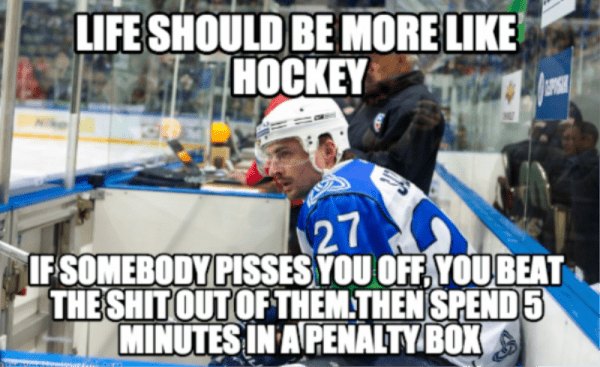The image is a meme featuring a photograph from a hockey game. It depicts a hockey player wearing a blue and white jersey with the number 27 and a white helmet, sitting inside the penalty box. Behind the glass enclosure of the penalty box, a person in a jacket (possibly security or a coach) can be seen, along with some desks with computers, indicating the organized environment of the arena. The stands are filled with spectators, and banners can be seen in the background, highlighting the lively atmosphere of the hockey game. Overlaid on the image is text in white, with the top part reading, "Life should be more like hockey," and the bottom part continuing, "If somebody pisses you off, you beat the shit out of them, then spend five minutes in a penalty box." This meme humorously suggests adopting the hockey culture of dealing with frustrations through brief, aggressive confrontations followed by short penalties.